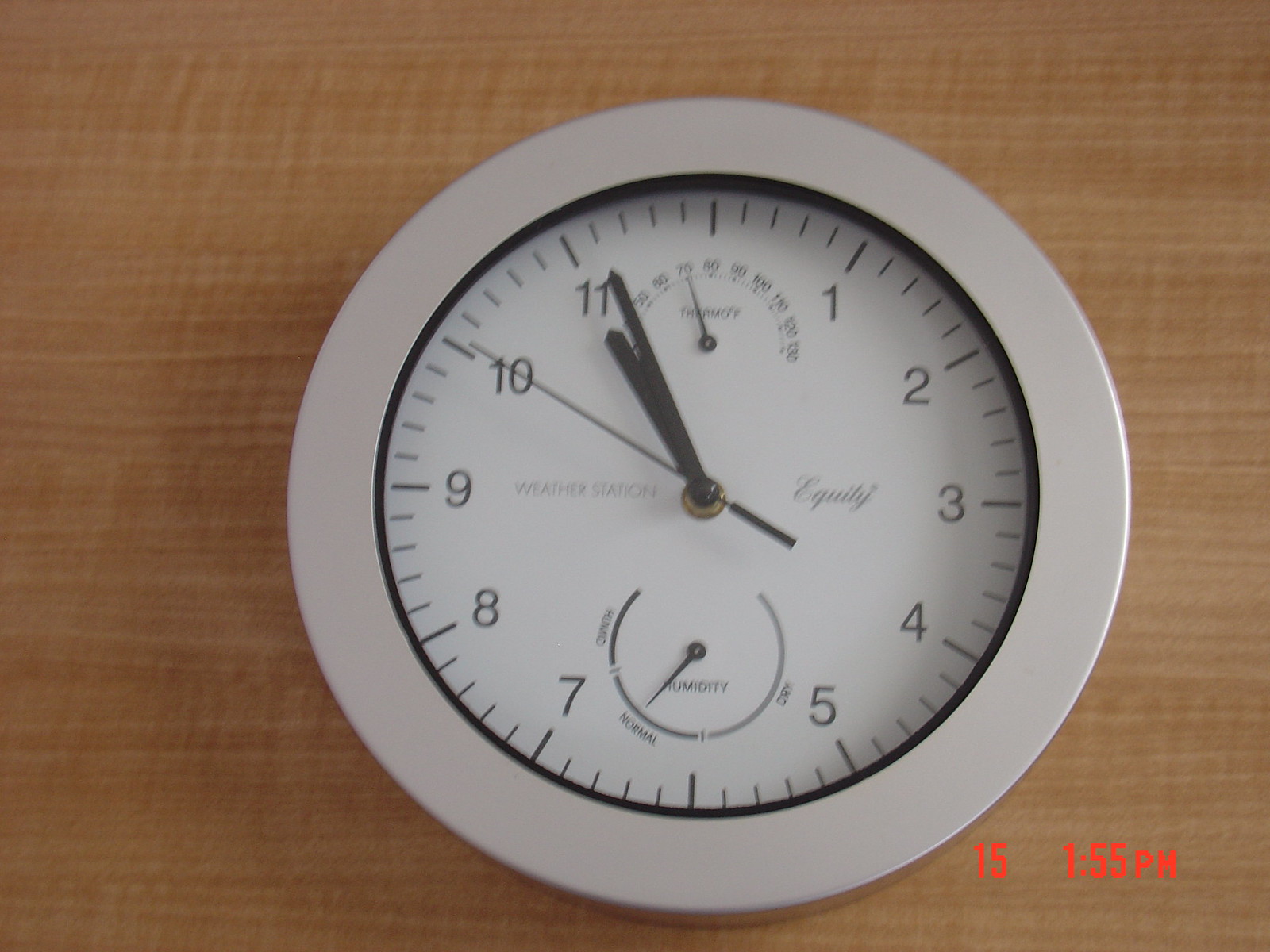The image depicts a round, white wall clock prominently positioned against a background of tannish-colored wood with visible grain patterns. The clock itself is a weather station, labeled "Equity," featuring a large white face with black markings and numbers, excluding the 12 and 6. The clock's black hands, including the second hand, indicate a time of approximately 10:56:50.

Within the main clock face, there are two additional smaller dials for measuring temperature and humidity. The top dial, a thermometer, displays a range from 50 to 130 degrees Fahrenheit, with the needle pointing to around 70 degrees. The bottom dial, a humidity gauge, includes segments labeled "humid," "normal," and "dry," with the needle positioned in the "normal" range. The digital photo also features a timestamp in the bottom right corner reading "1:55 P.M." along with the number "15" farther to the left.